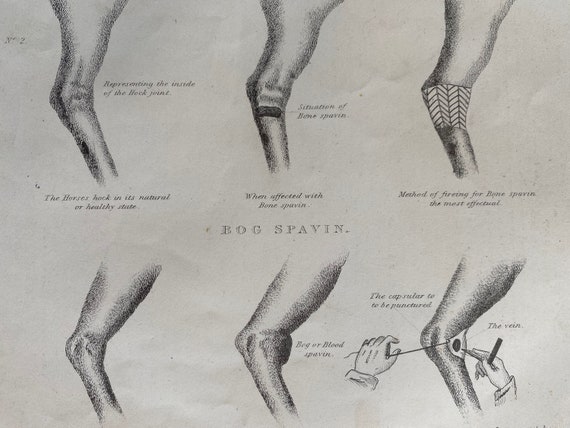The rectangular black and white illustration depicts six bent horse legs, carefully detailed to show various types of first aid applications. The legs are arranged such that they resemble the anatomical structure of a deer's legs, from the upper thigh to the lower leg. The vintage-style image is faded, giving it a grayish color and a somewhat worn appearance.

In the center of the illustration, the words "bog spavin" are clearly legible, referring to a specific equine condition. Above this, there is a faded but readable note: "The horse’s hock in its natural healthy state," clarifying that the artwork represents the legs of a horse. 

Each leg depicted has a different form of treatment:
- The upper center leg is shown with a bandage or band-aid applied.
- The lower right leg features two hands demonstrating the process of suturing an injury with a needle and thread.

The detailed, albeit worn-out illustration, serves as an educational display, likely from a vintage veterinary guide, emphasizing the diagnosis and treatment of horse leg conditions such as bog spavin.